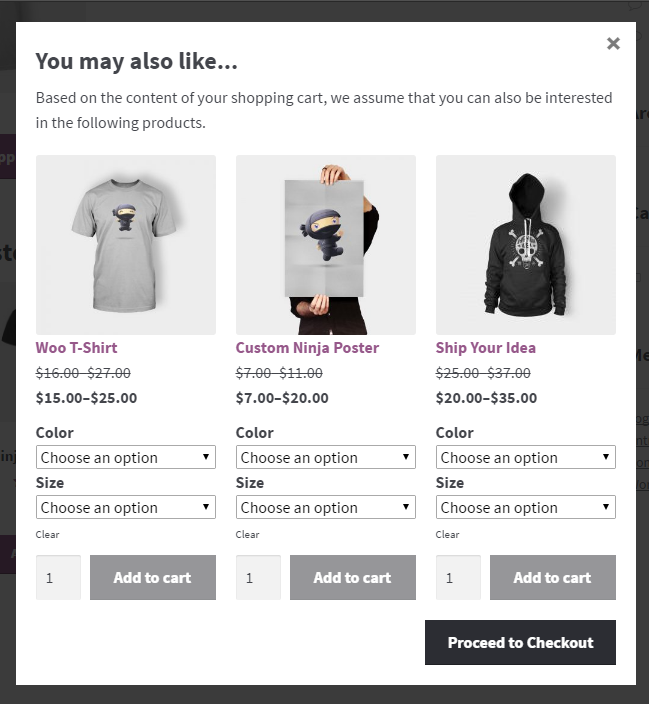This website displays a selection of recommended products based on the contents of the user's shopping cart. The suggested items include a "Woo T-shirt" priced between $15 and $25, a "Custom Ninja Poster" ranging from $7 to $20, and an item labeled "Ship Your Idea" which costs between $20 and $35. Each product listing features drop-down menus for selecting color and size options, a clear button, a quantity selector starting at one, and an "Add to Cart" button. There is also a "Proceed to Checkout" button for finalizing purchases.

The Woo T-shirt is gray and features a small black cartoon ninja character. The Custom Ninja Poster has the same ninja design. The "Ship Your Idea" hoodie is black, adorned with a white skull and crossbones design, and includes white drawstrings.

Text throughout the website is primarily black, except for the product names which are displayed in purple. The "Add to Cart" and "Proceed to Checkout" buttons are white, with the former encased in a gray border, and the latter featuring a black background. The entire page is outlined by a black border, and individual buttons are similarly trimmed with gray. All these elements are designed to create a clear and cohesive user experience.